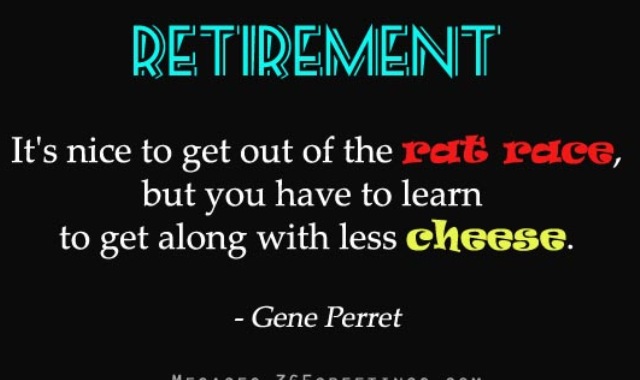The image is a black rectangular card bearing an inspirational quote. At the very top is the word "Retirement," spelled out in large, aqua blue letters with black borders, creating a 3D effect. Below, the quote begins in white text with the line, "It's nice to get out of the," followed by "rat race" in larger, bold red text. The next line continues in white, stating, "but you have to learn to get along with less," while the final key term "cheese" is emphasized in larger, bold yellow text. The quote is attributed to Jen Parrott, whose name is printed in white at the bottom of the card. The layout includes some additional, partially visible text below the attribution.